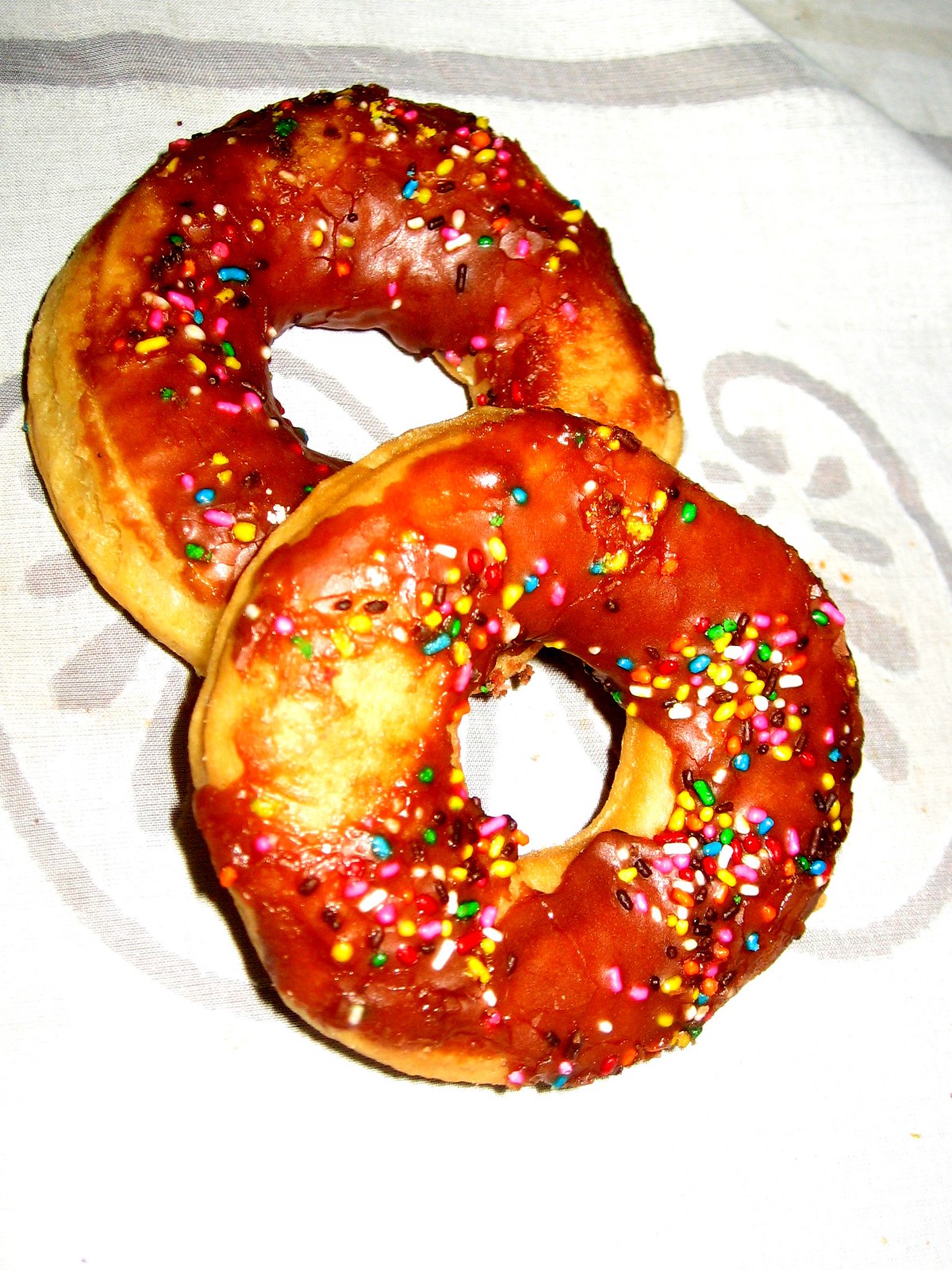This photograph showcases two regular, tan doughnuts with light brown frosting, perched on a white kitchen towel adorned with blue and grey markings. The doughnuts are generously sprinkled with an array of colorful sprinkles, though some frosting is bare, exposing the dough beneath. Notably, a few of the sprinkles are clumped together. One doughnut slightly overlaps the other, partially obscuring it. The top doughnut features a lightly burnt section, adding character to its appearance. The intricate details and tempting appearance of these round, hole-in-the-center doughnuts make them look particularly appetizing.